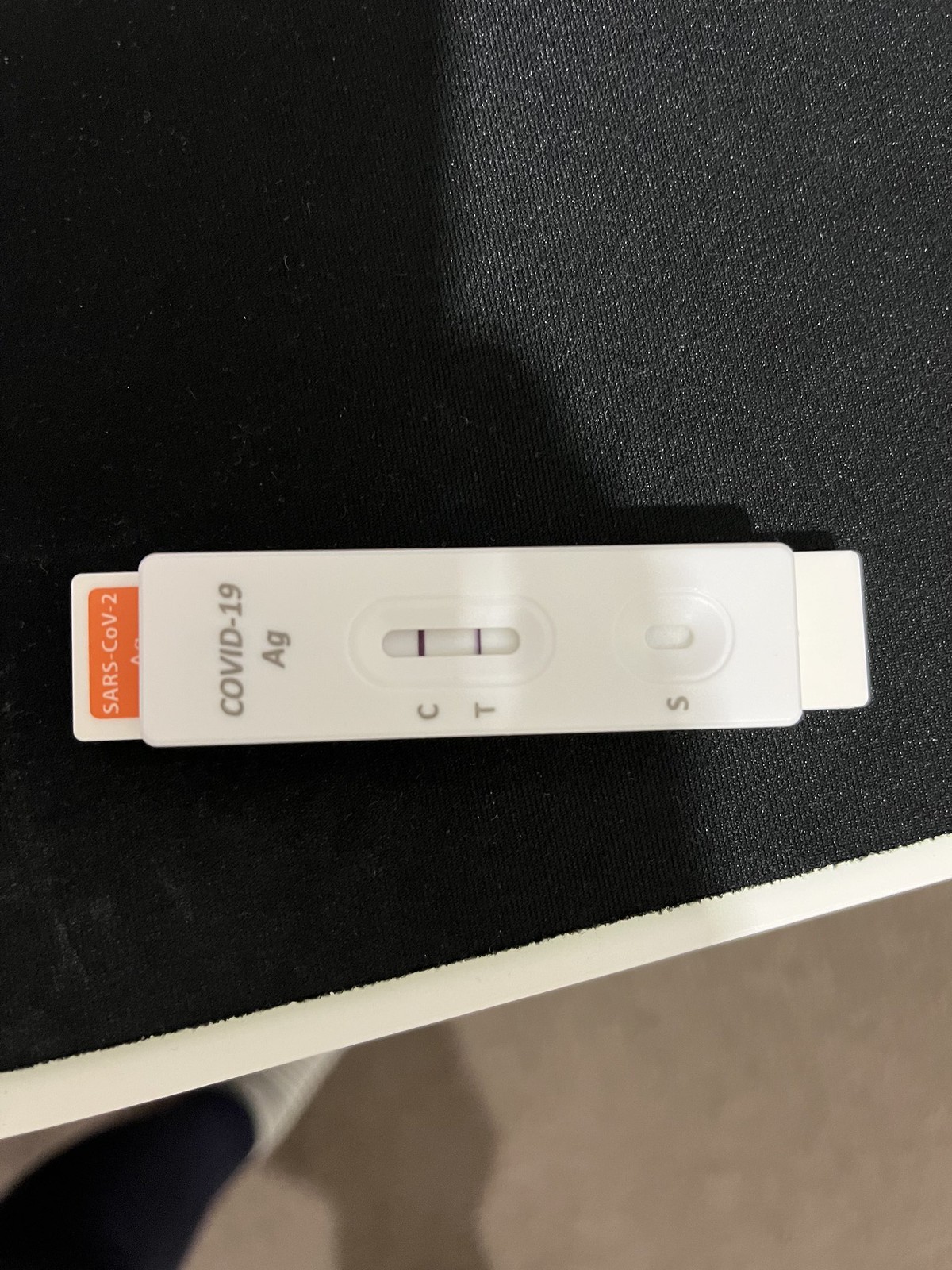In this detailed close-up photograph, the focal point is an in-home COVID-19 antigen test. The test device, primarily white in color, prominently displays the words "SARS-COV-2" in white letters against an orange background on the left side. Adjacent to this, the text "COVID-19-AG" is clearly visible. 

At the center of the device is a small viewing window displaying the indicators "C" and "T," with two lines visible, signifying a positive result for COVID-19. On the far right of the device are the abbreviations "S" and "L." 

The design includes a small circular well on the right-hand side, where a sample solution, derived from a nasal or throat swab, is deposited. Within a few seconds, the results manifest as lines in the window, with both lines indicating a positive result for the virus, and a single line at "C" indicating a negative result.

The background highlights a blackish felt-like tabletop surface, adding a contrasting backdrop to the white test device. In the bottom left corner, a partial view of what appears to be a human leg is visible, slightly emerging into the frame.

Overall, this image meticulously captures the essential details and instructions related to the COVID-19 antigen test, emphasizing its function and reading procedure.